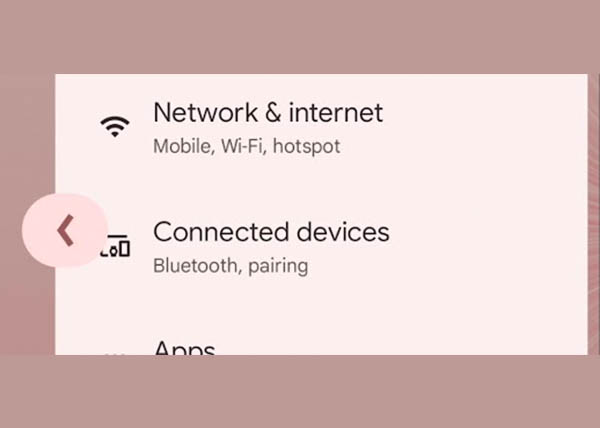The image features a horizontally elongated tan-colored rectangle, overlaid by a smaller, centrally placed, peach-colored rectangle at the top. On the left side, a circle containing a left-pointing backward arrow overlaps with the background. This arrow is in a pink shade that differs from the surrounding pinks, and it is slightly darker, matching the tan-pink hue of the background.

Within the smaller peach rectangle, the content includes text in black or gray font that reads: "Network and Internet, Mobile, Wi-Fi, Hotspot, Connected to Devices, Bluetooth Pairing," followed by a partially visible word "Apps" that is cut off halfway. The background of this inner rectangle is light pink, providing a gentle contrast to the tan-pink surroundings.

The image exhibits some blurriness around the lettering at higher resolutions, although it remains clear and easily readable when viewed at its original size. This composition highlights a minimalist design approach with a focus on service options and connectivity, set against a soft, pastel-colored palette.